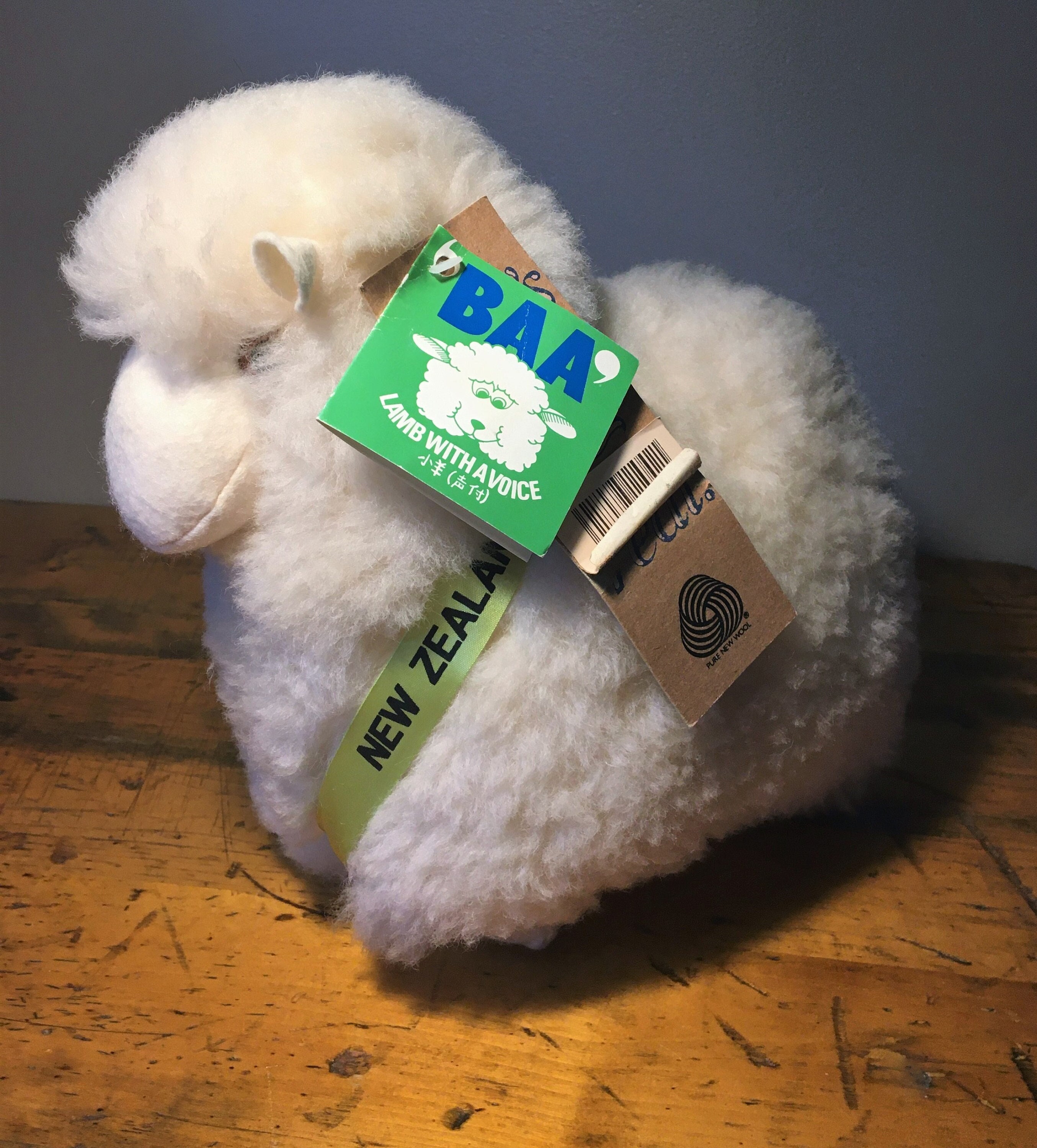This photo showcases a small, fluffy, cream-colored stuffed lamb toy sitting on a scratched, wooden surface, likely a desk. The lamb has a pillowy face made of white felt material, with its black eyes partially obscured by its fur. It features round, folded ears. The lamb is adorned with a green ribbon around its neck that says "New Zealand" in black text. On its head, there are two tags attached: a square tag with blue text reading "Baa" and an image of a lamb with the phrase "lamb with a voice," and a longer, brown rectangular tag with a peeling barcode sticker and a wolf symbol. The background of the image is dark gray, giving a slightly murky effect, with a light focus on the toy itself.